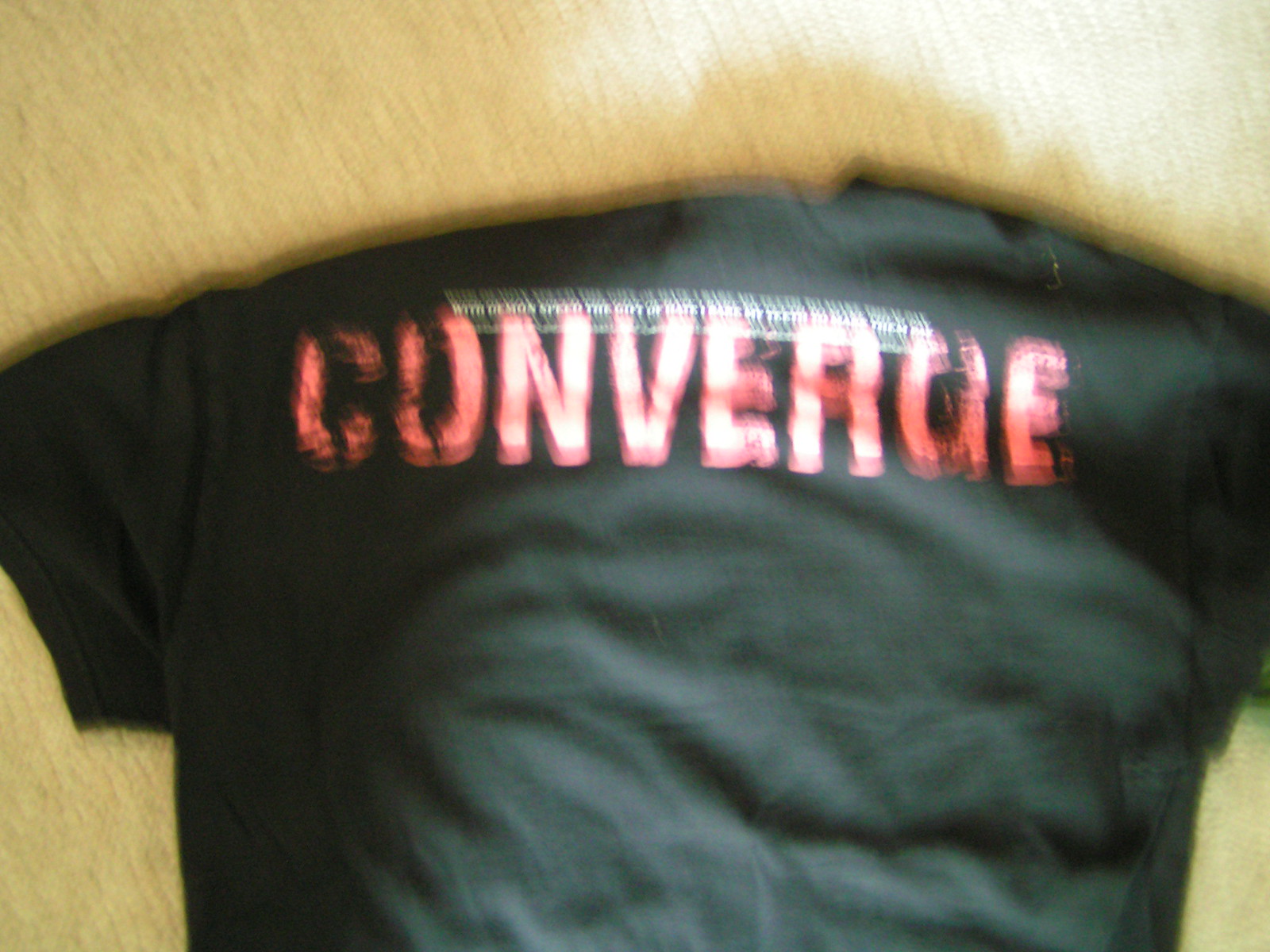In this very blurry image, a black, short-sleeve t-shirt is shown laying wrinkled on a light beige or tan flooring. Dominating the back of the t-shirt is the word "CONVERGE," spelled out in capital letters with a light reddish color that appears worn, fading, and somewhat wispy, adding a slightly eerie effect. Overlaying the red CONVERGE text is a smaller, white text that is partially decipherable, including phrases such as "WITH demon speed," though the photo's blurriness makes the full text challenging to read. The shirt is illuminated by a bright white light shining directly down its center, casting shadows towards the top right corner.